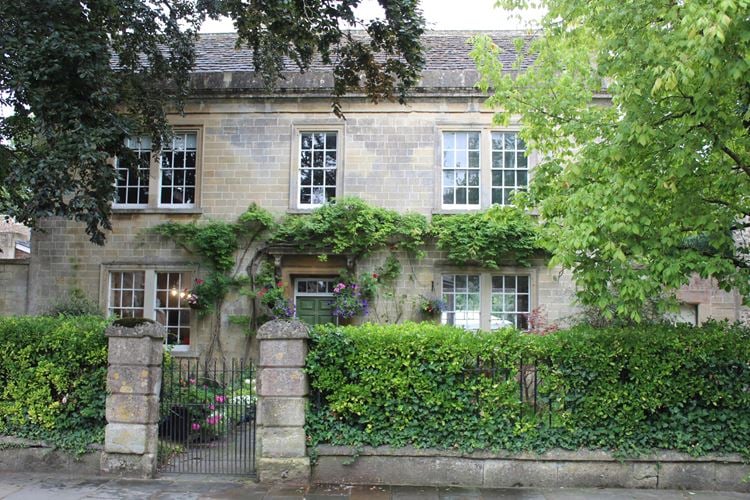The image depicts the exterior of an older, two-story brick house located in a typical neighborhood. The front yard is enclosed by a small black gate flanked by two stone columns. The house, constructed of brown brick, features a total of nine slender windows configured in pairs: two pairs on the top left and right, two pairs on the bottom, and a single window directly above a green door. Vines embellish the top of the green door and spread along the doorway and nearby windows. The roof of the house is a dark gray to black shade. Two trees are present in the front yard; the one on the left has darker green leaves, while the one on the right has brighter green leaves. Additionally, bushes partially conceal another black gate. Greenery, including a bushed fence and various plants, adds to the house's charm, and the sky appears cloudy on the day the photo was taken.